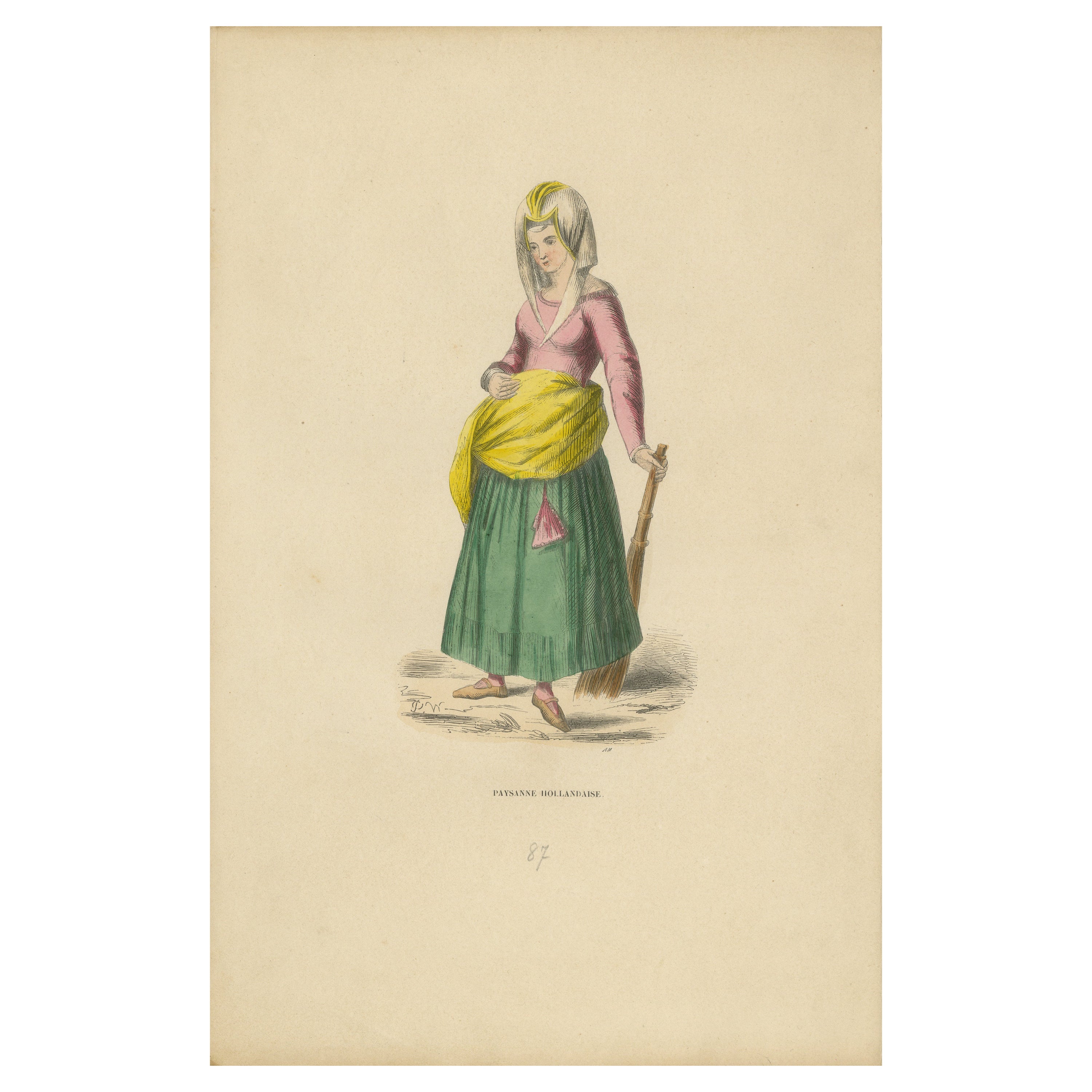This detailed drawing features a woman in traditional attire. She is wearing a pink blouse with a collar and a long flaring green skirt that extends down to her legs. Draped around her waist is a yellow cloth, giving her a layered look. On her head, she wears a headdress or scarf that extends below her neck and has a yellow outline. The illustration captures her holding an old-fashioned wooden broom with both hands, her right arm positioned around her waist and her left arm supporting the broom down to the ground.

The artwork appears to be somewhat aged, with faded coloring on a light pinkish-beige background. The text beneath the woman reads "Payson, Hollandese," followed by the faint number "87," although this text is somewhat blurry. The drawing is approximately the dimensions of a page in a magazine and gives off a historical vibe, possibly depicting a person from an earlier time period. The overall impression suggests a mix of traditionalism and timelessness in the woman's appearance.